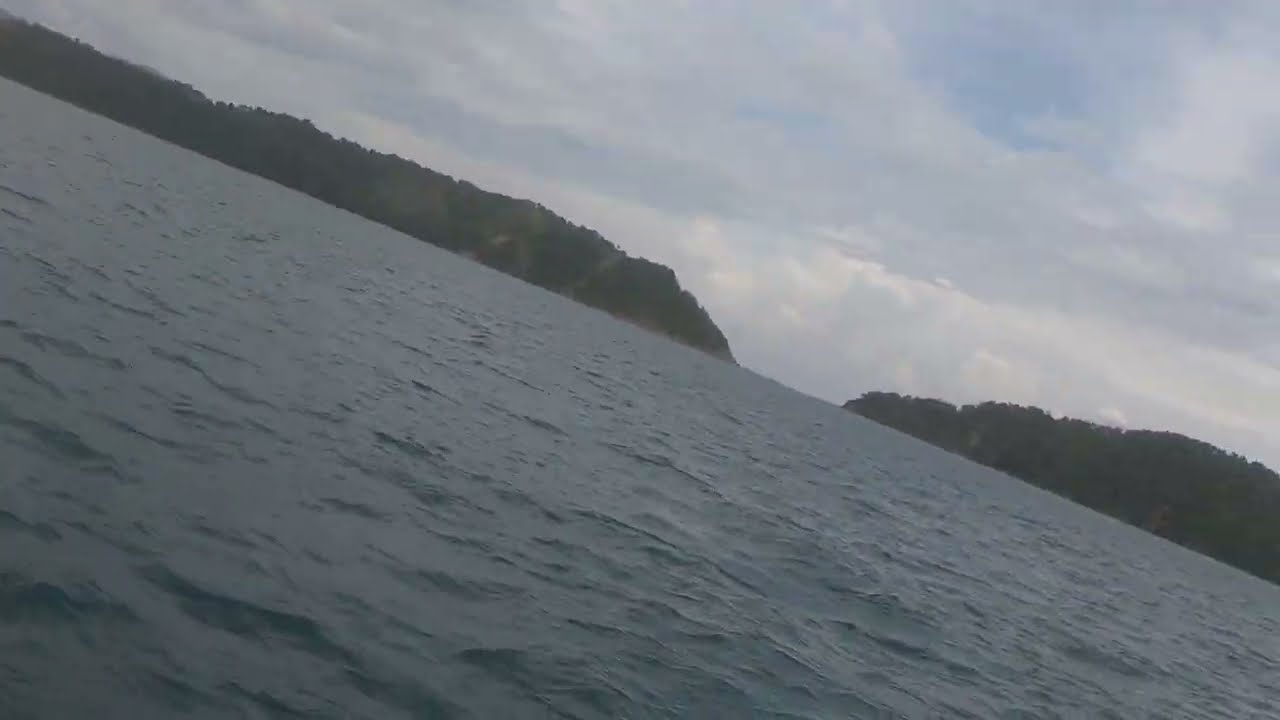The image depicts an expansive outdoor scene centered on a large body of slightly rippled water, primarily exhibiting a grayish-blue hue. The water flows toward the background where it meets two large hills or mountain ranges densely covered with green vegetation. The hills, nearly identical in size and elevation, are split by the continuation of the water itself. The sky above is overcast with predominantly gray and white clouds, yet patches of blue sky can be seen breaking through. The perspective of the photo is slightly angled to the right, giving an impression of both an overhead and a sideways view, enhancing the grandiosity of the scene. The landscape is devoid of any man-made structures, highlighting the untouched natural beauty of the area.